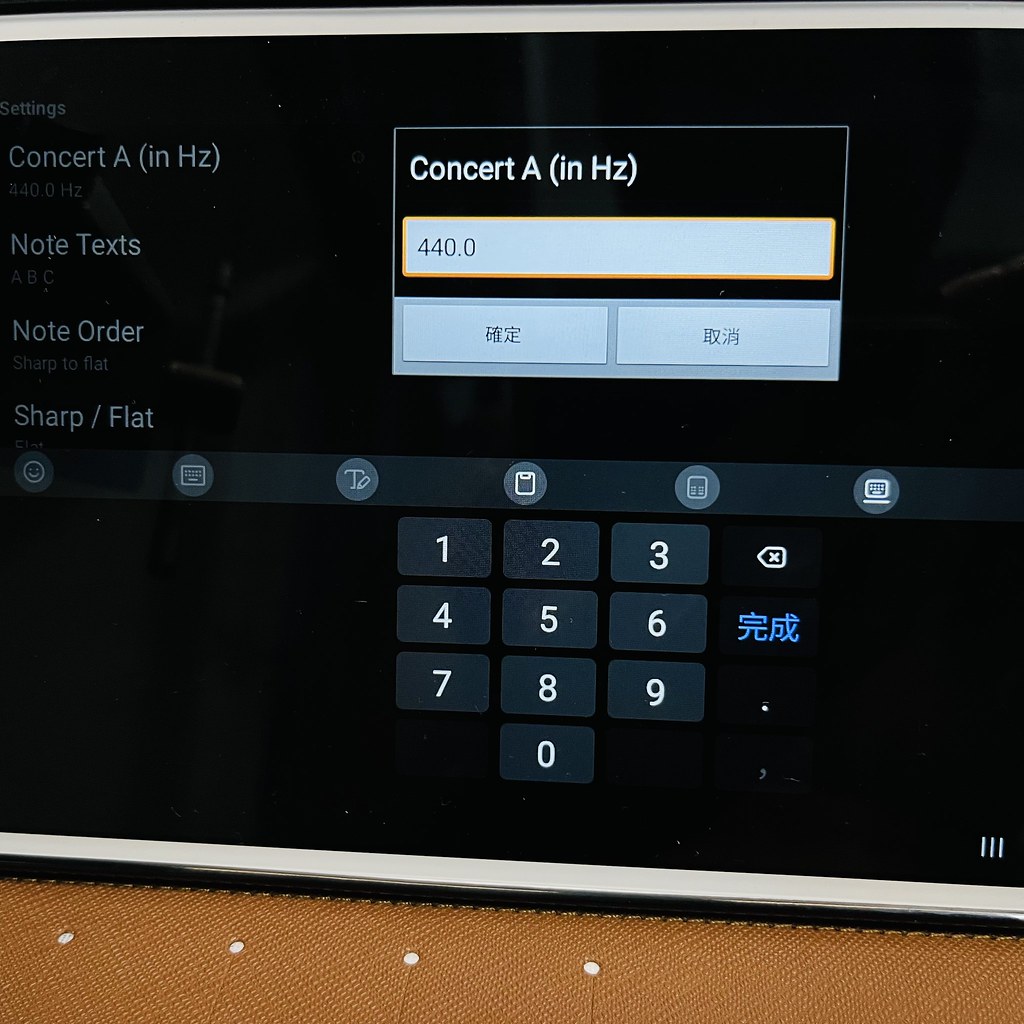The image shows a close-up of a digital screen, possibly from a tablet or a cell phone. The screen has a black background with predominantly blue and white text. At the very top, it says "Concert A in Hz" and "440.0", which indicates the frequency of the A note in Hertz. Below this header, there are two clickable white rectangles containing Chinese characters. The middle section of the screen has text including "Settings," "Concert A in Hz," "Note Text," "Note Order," and "Sharp/Flat." To the left center, there’s a box with "Concert A (Hz)" in white. Following this, there is a blue box displaying "440.0." The bottom portion of the screen resembles a calculator with a number pad layout, showing numbers 1 through 9 arranged in a 3x3 grid, with the number 0 at the center bottom. To the right of the number pad, there is an "X" and additional Chinese characters. At the very bottom, the screen appears to be attached to a brown base, possibly made of leather.